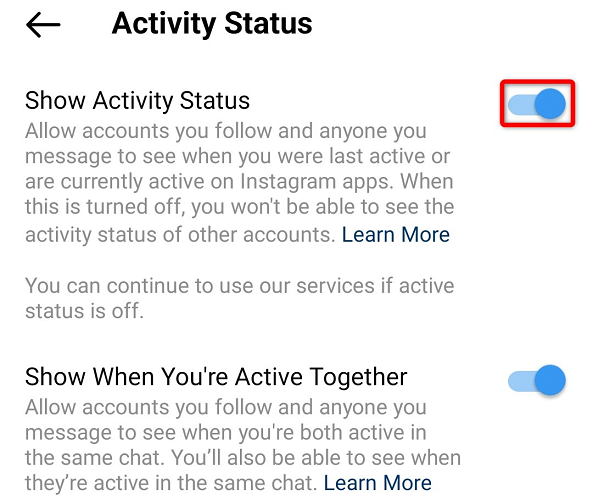The top left corner of the image features a left arrow icon. To its right, there's a section titled "Activity Status," followed by a blue toggle switch with a red border labeled "Show Activity Status." 

Below this, detailed in clear text, is an explanation: "Allow accounts you follow and anyone you message to see when you were last active or are currently active on this app. When this is turned off, you won’t be able to see the activity status of other accounts." There is a note in grey text stating, "You can continue to use our services if active status is off."

Further down, there's another option titled "Show When You're Active Together," with text explaining: "Allow accounts you follow and anyone you message to see when you're both active in the same chat. You'll also be able to see when they’re active in the same chat." An option to "Learn More" is available as well.

The image has a white background with minimal other visible elements, and there is a small text display showing "052."